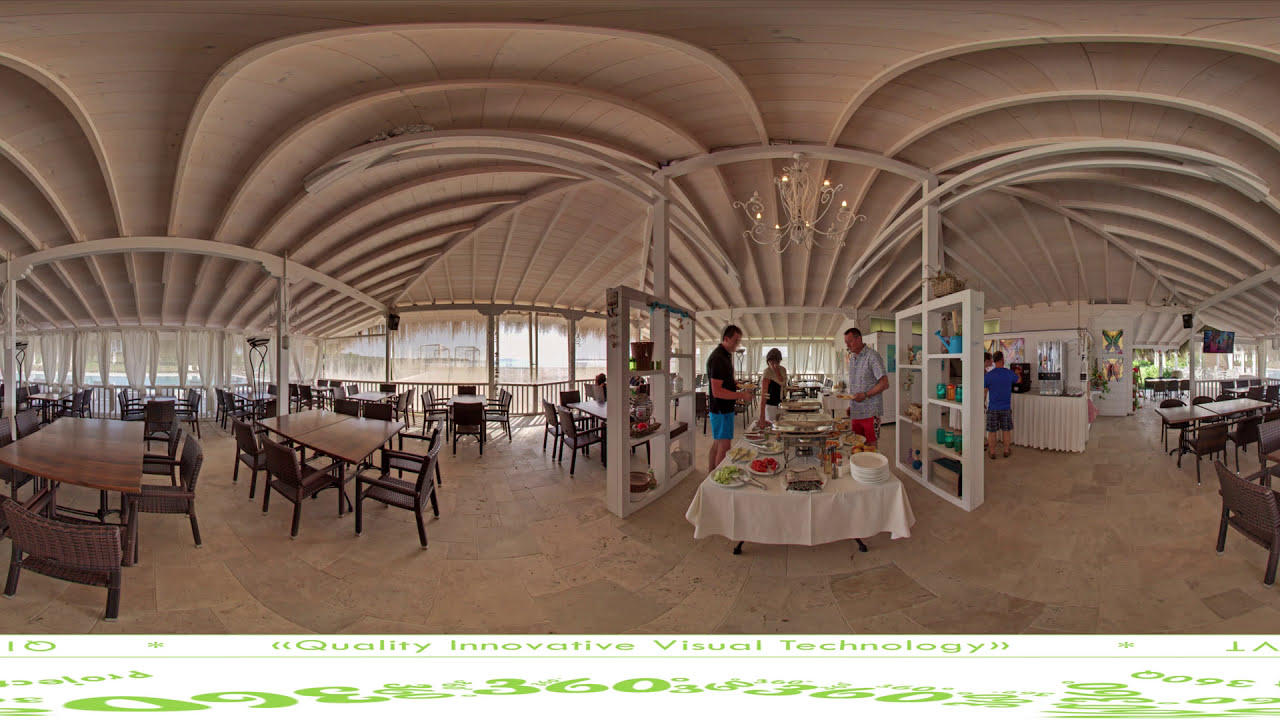The image depicts a spacious, indoor dining area that seems to be set up for an event or buffet-style meal. The ceiling is notably adorned with unique, closely-knit semicircular wooden carvings, lending an artistic touch to the ambiance. On the left side of the image, several windows with white curtains offer a view to the outside, where a blue swimming pool is faintly visible. Below the windows, brown rectangular tables are paired with wicker chairs, contributing to the cozy yet elegant atmosphere.

Central to the image is a long table draped in a white tablecloth, laden with a variety of foods and a neatly stacked pile of white plates. Surrounding this buffet table are three individuals—a man in blue shorts and a black shirt, another man in light blue shorts and shirt, and a woman—each intently focused on the food offerings. Above this scene, a white chandelier hangs from the intricately designed ceiling, illuminating the area.

Flanking the buffet table are two white bookshelves or cabinets, each with multiple square compartments holding various items. On the right-hand side, another group of people can be seen either paying or ordering from a smaller table. The background of the image reveals more brown tables and chairs spread across a light beige, square-tiled floor. Additionally, a banner reading "Quality, Innovative, Visual Technology" with a 360-degree camera shot indicator is displayed along the bottom width of the image. This caption blends the variety of details captured in each individual description, creating a coherent and detailed portrayal of the scene.